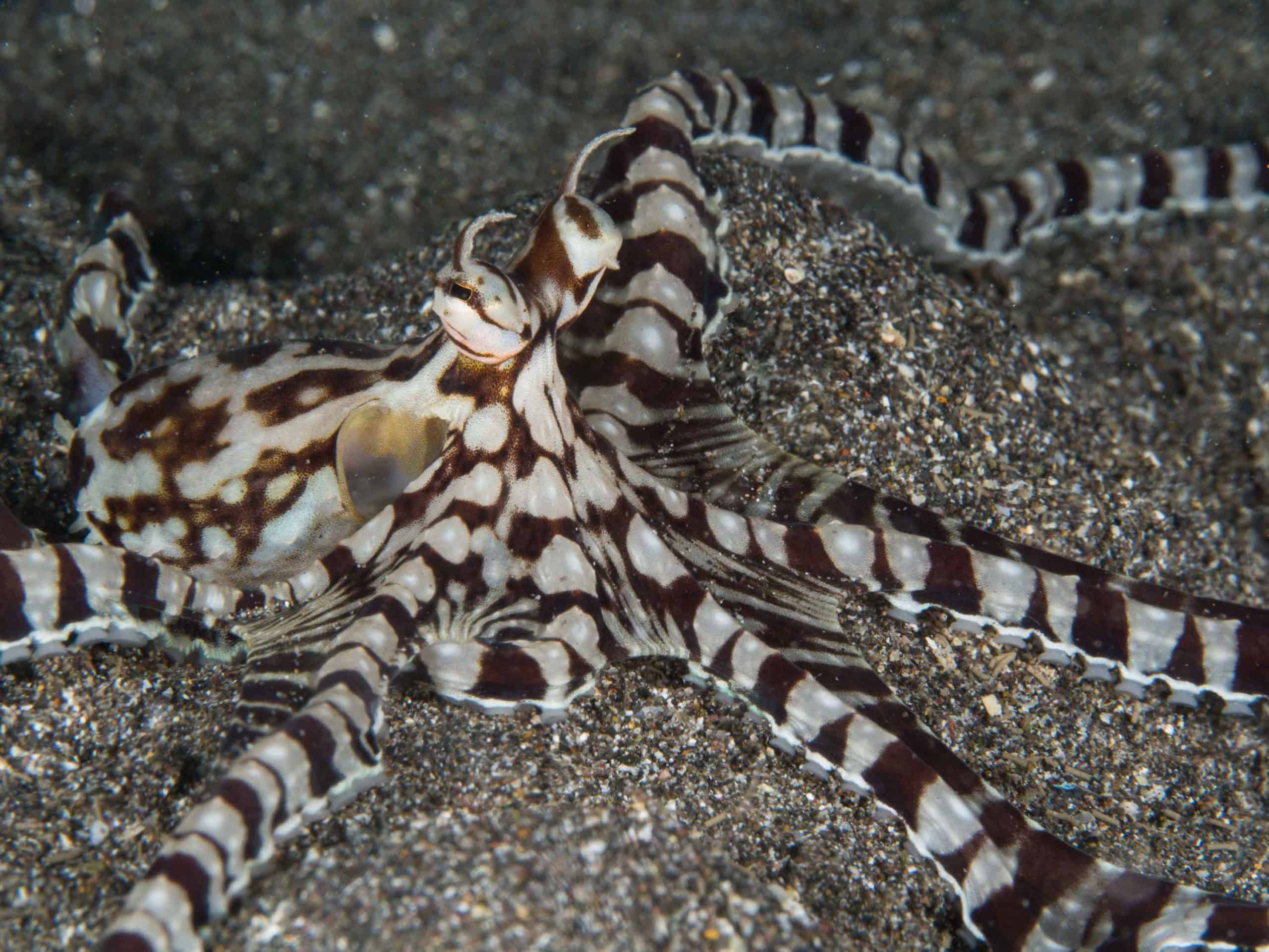The image depicts a close-up view of a striking octopus nestled on the sandy seafloor. The sand comprises large and fine particles interspersed with tiny white, black, and gray stones, setting a textured background. The octopus itself dominates the picture with its body and head located towards the left side, displaying a mix of dark brown and white stripes and spots. Its long, thin tentacle arms, six of which are spread out almost snake-like across the sand, lack visible suckers in this top-down view. The octopus's bulbous head can be seen clearly, along with its eyes and antenna-like structures that add to its marine essence. Light, shadows, and natural underwater highlights accentuate the amphibious creature, contributing to the vibrant, eco-conscious scene that underscores themes of marine life and environmental awareness.